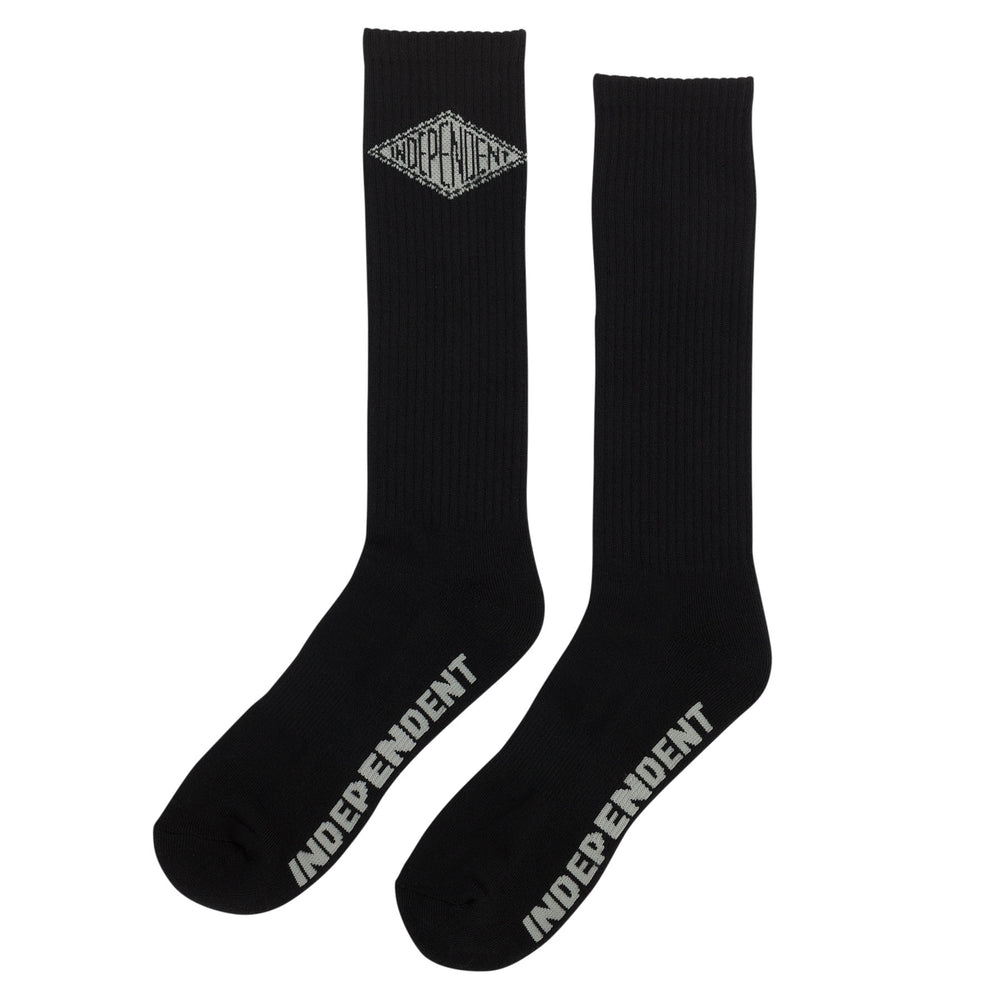This is a highly detailed image of a pair of black socks presented against a white background. The socks appear to be calf or knee-length and are identical in design. Each sock features the word "independent" written in white on the left side of the foot. Additionally, the right sock displays a gray diamond-shaped logo near the top, containing the word "independent" in a stylized black font. In this logo, the letters 'IN' at the beginning and 'NT' at the end are notably smaller, with the central 'DEPEND' portion in larger letters that stretch the length of the diamond's height. Overall, these are straightforward black socks with notable branding details.